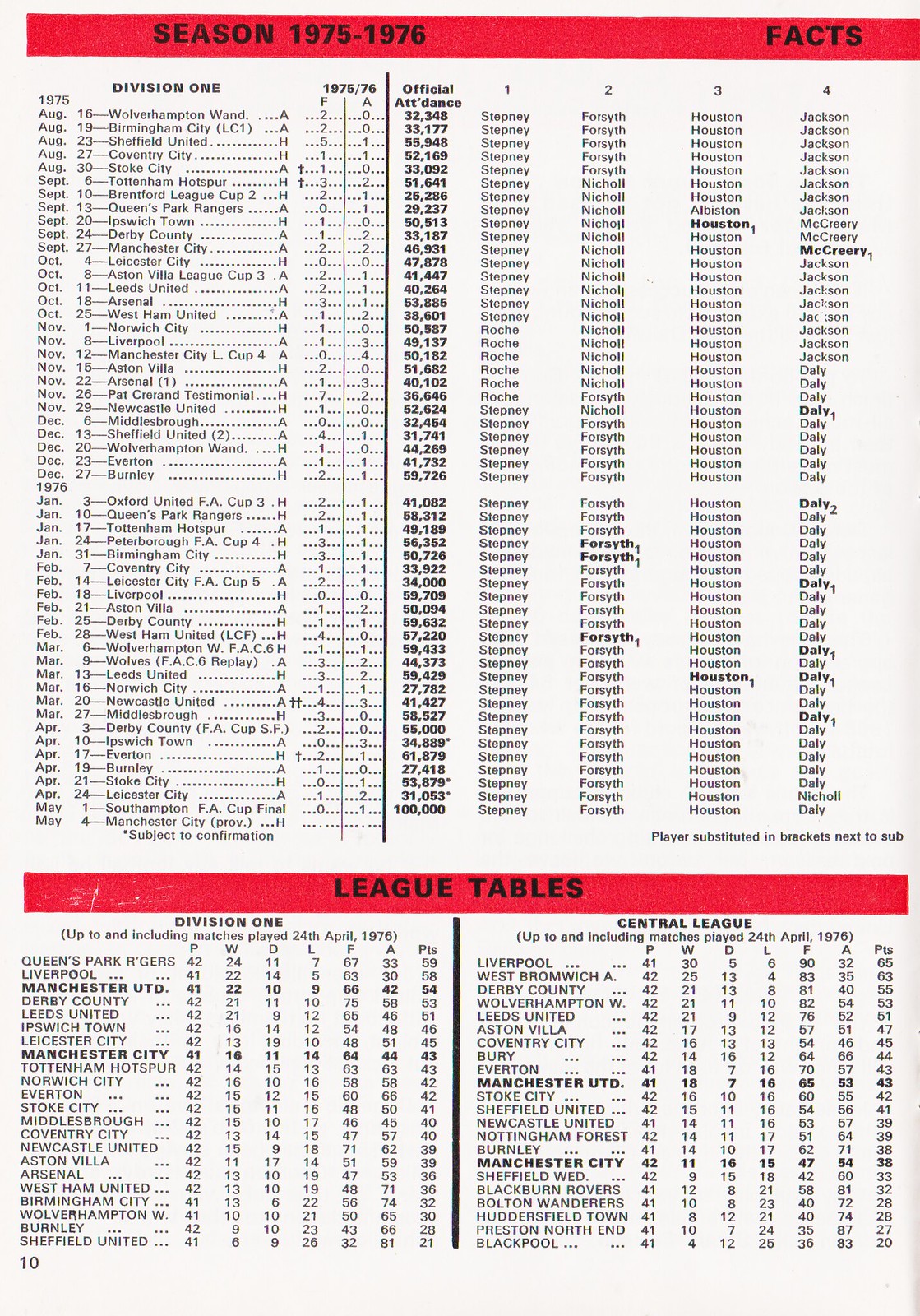This image appears to be a page from a soccer magazine, specifically page 10, detailing a range of statistics from the 1975-1976 season. At the top of the page, a red text box with black, all-caps lettering states "Season 1975-1976 Facts." Below this heading is a detailed table labeled "Division 1," listing various dates, cities or teams, and official attendance figures. Further down, another red banner with black, all-caps text reads "League Tables." This section features two side-by-side tables: the left one under the heading "Division 1" and the right one titled "Central League." Both tables include statistical columns marked PLDLFA and Points, offering comprehensive data for the teams of that period. The layout is heavily text-oriented, focusing on the detailed presentation of soccer statistics.